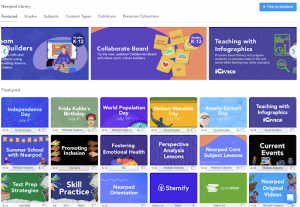The image showcases a slightly wider-than-tall layout of a web page, roughly 30% wider. The image is small and much of the text is indistinct, so a detailed description follows. At the top left corner, there is a two-word title in gray text set against a white background. Directly below this title are six horizontal menu options extending from left to right. In the upper right corner, a prominent blue button with white text is displayed.

Beneath the menus, there are three horizontal rectangles predominantly featuring a purple hue. Navigation arrows, colored blue, flank these rectangles, indicating the presence of additional content beyond the displayed three.

Occupying about 60% of the lower section of the image is a grid of colorful squares. These squares are varied in color, including shades of blue, green, purple, yellow, and black. The grid is arranged in a six-by-three formation, totalling 18 squares. Each square is adorned with white text that labels the respective links or functionalities they represent.